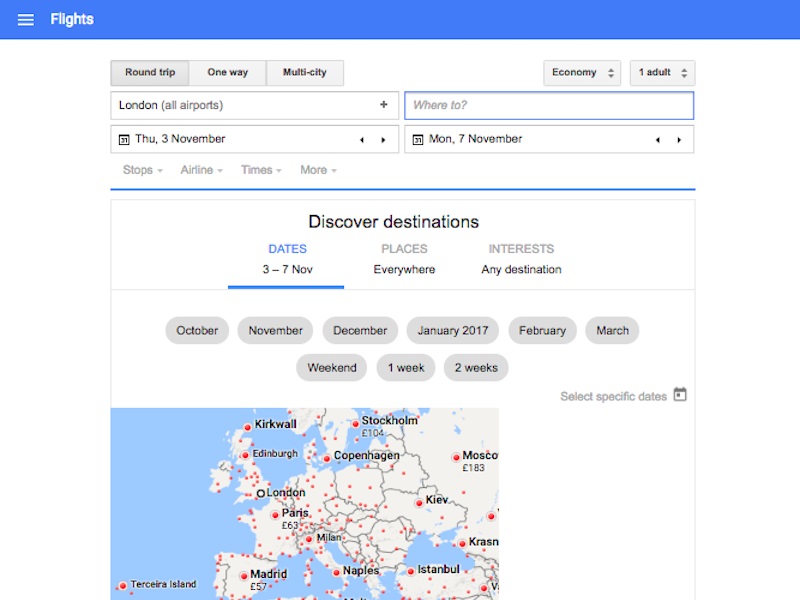The image depicts a flight booking interface originating from London, showcasing various destination options primarily across Europe. The user's search dates span from November 3rd to November 7th. Prices are only partially visible, with some examples being €63 for Paris and €57 for Madrid. This booking site supports multi-city and round-trip options, displaying round-trip prices in economy class for one adult. The interface features a distinctive blue border at the top, with the remaining sections in white.